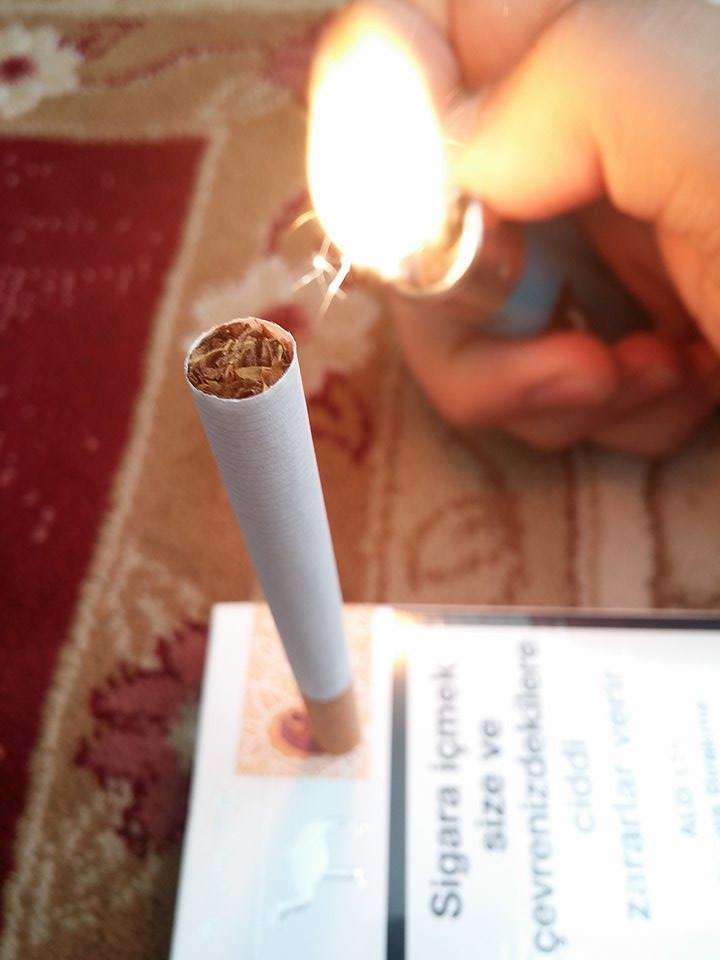This close-up photograph captures a moment of igniting a cigarette. The focal point of the image is a cigarette standing upright on a white surface, which features black lettering in a non-English language, "Cigarra Ikmek Size VE Kovren Sedekeler." The cigarette, with its white paper and tobacco-filled open end facing up, has a yellow-tipped filter resting on the surface, possibly a book or piece of paper. The person’s right hand, positioned in the top-right corner of the photo, is holding a round, blue lighter, with their thumb pressing down on the ignition. The lighter's bright flame, which dominates the upper part of the image, is directed toward the cigarette. Surrounding the scene, a patterned rug frames the composition with a white flower visible in the top left and a portion of a pink flower beneath the surface on which the cigarette stands.